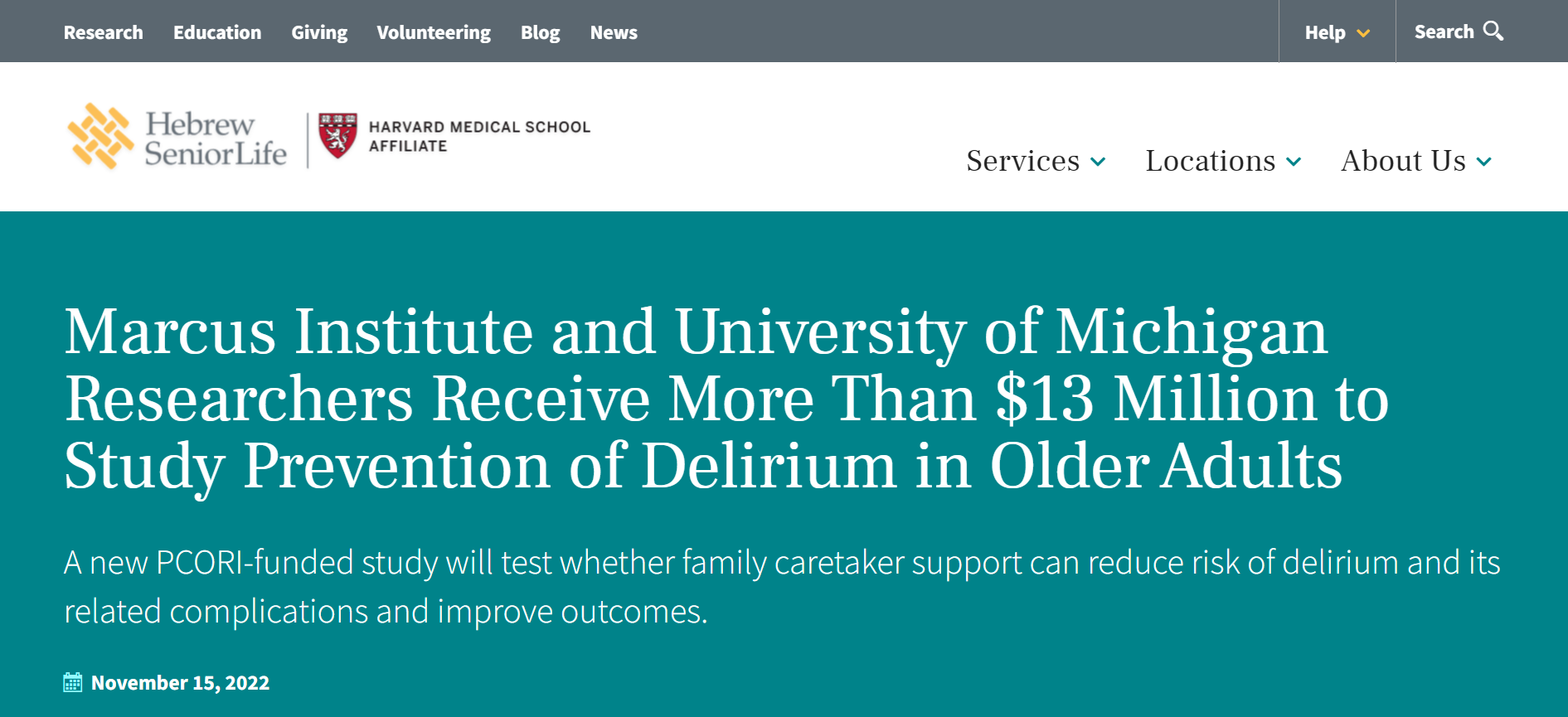This is an image of a website featuring a detailed layout with sections dedicated to various topics. At the top, there is a grey navigation bar with white text. The top left corner includes navigation options such as "Research," "Education," "Giving," "Volunteering," "Blog," and "News." To the right of these options are two additional features: "Help," which is a dropdown menu, and a "Search" function accompanied by a magnifying glass icon.

Below the navigation bar, the website's name "Hebrew Senior Life" is prominently displayed next to a grid-like yellow logo, separated by a vertical line. Adjacent to this, the text "Harvard Medical School Affiliate" is shown alongside the Harvard badge.

Further to the right, several more dropdown options are visible, including "Services," "Locations," and "About Us," the latter marked with a small blue arrow indicating additional choices.

A teal-colored section below these elements highlights a significant announcement: "Marcus Institute and the University of Michigan researchers received more than $13 million to study prevention of delirium in older adults. A new PCORI-funded study will test whether family caretaker support can reduce the risk of delirium and its related complications and improve outcomes."

In the bottom left corner of this announcement, a white calendar icon is displayed with the text "November 15, 2022."